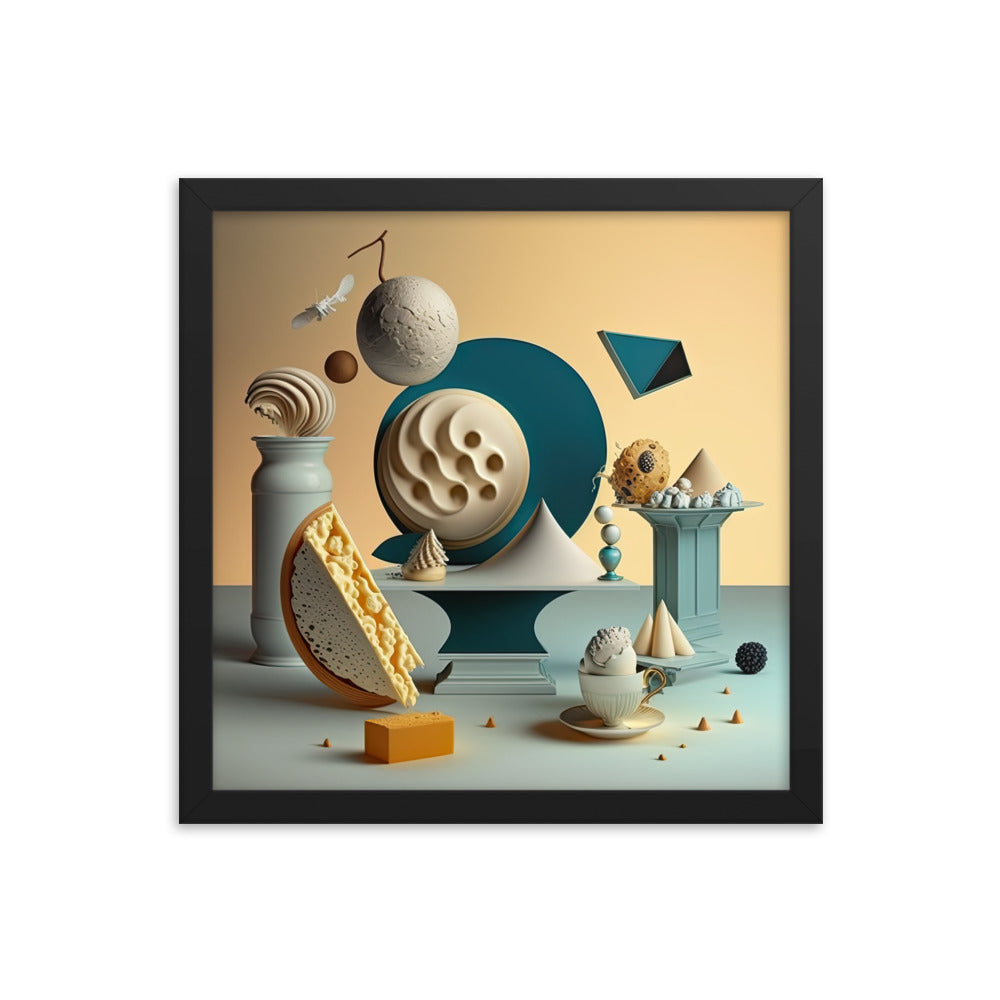This framed computer-generated artwork, reminiscent of a surrealist painting with Dali influences, showcases a vivid, almost claymation-like scene. Dominated by a light mustard yellow at the top, the image features various food-inspired shapes rendered as sculptural forms. A bowl of mac and cheese halved, a teacup and saucer possibly filled with ice cream, and a bottle of milk spilling its contents are central elements. The bottom left displays a crescent-shaped, yellow cheese cutout, while teal-colored bases and pillars stand against a white floor. Triangular shapes scatter across the ground, and floating geometric forms punctuate the scene, adding to its dreamlike quality. The entire piece is encapsulated by a dark black frame, enhancing the striking, surreal contrasts within.